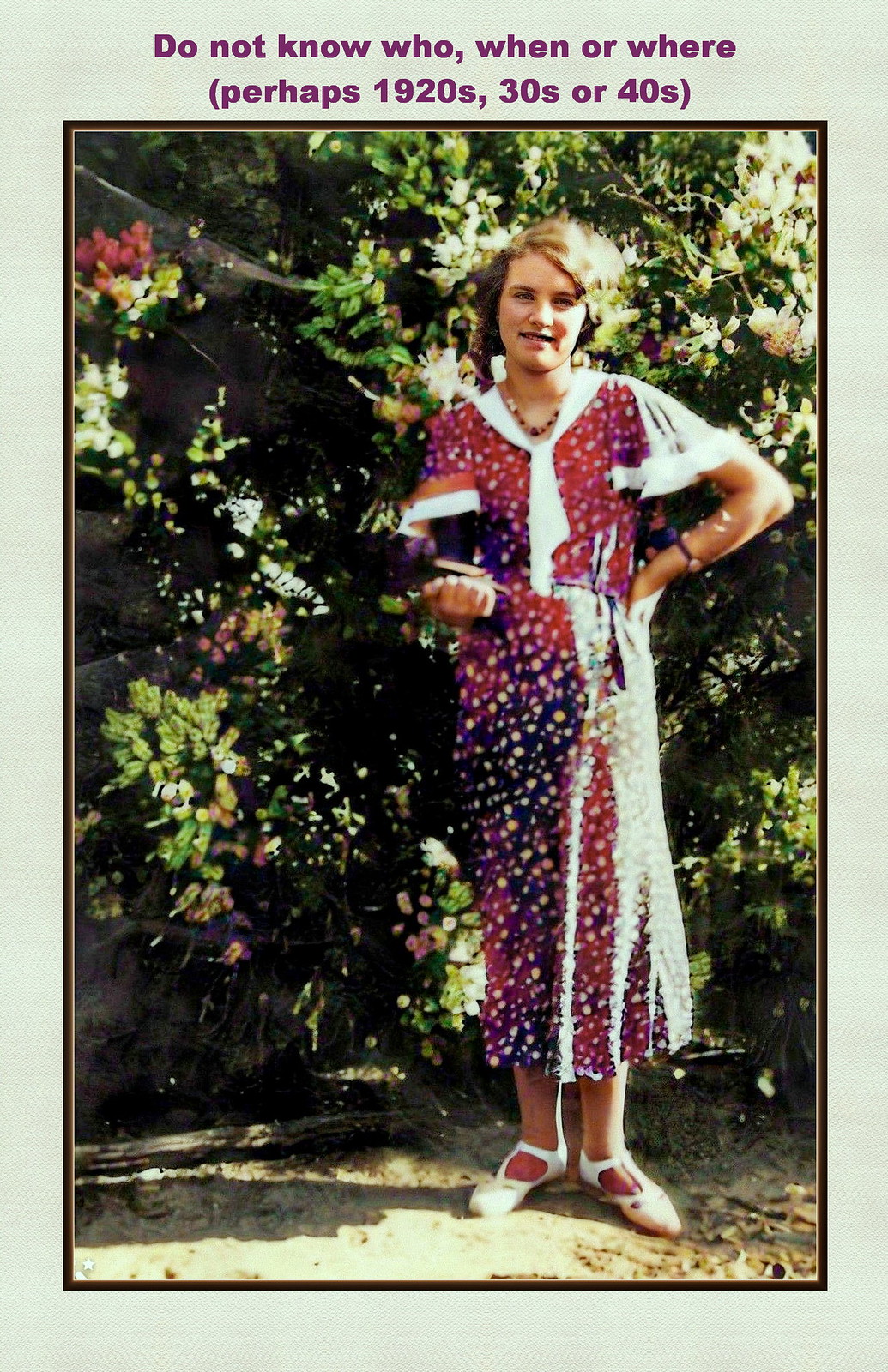The image captures a young woman with light skin and short, dark blonde to brown hair, standing in a vibrant flower garden. She is positioned in the right one-third of the frame, wearing a red or pink floral dress adorned with white and blue polka dots. Underneath her dress, she has a white undershirt and around her neck, she sports a red and white necklace that almost resembles a sailor's collar. Her white sandals are neatly aligned with her heels together and toes pointed outwards.

The woman’s pose is confident, with her left hand on her hip and her right hand holding an object, possibly a book, close to her side. Her facial expression is a smile directed at the camera. She wears a bracelet on her left wrist, adding a subtle touch of elegance. The backdrop is a lush display of flowering plants in a variety of colors including green, yellow, red, brown, and white, indicating it is daytime with ample natural light.

Encircling the image is a black border framed by a white or light blue background. At the top, red text reads: "Do not know who, when, or where (perhaps 1920s, 30s, or 40s)."